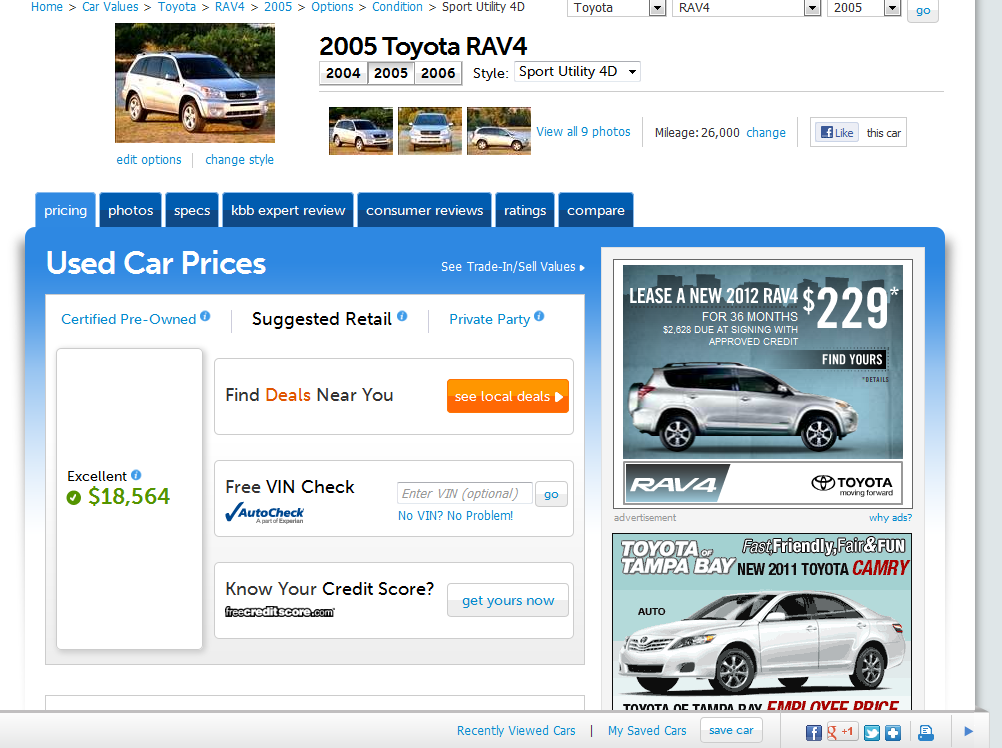**Detailed Descriptive Caption:**

This is a comprehensive screenshot from a car valuation website, specifically geared towards offering used car prices. Dominating the top-left corner of the webpage is an image of a silver SUV. Next to this image, in large, bold, black text, is the designation "2005 RAV4." Directly beneath this title, there are three clickable buttons labeled 2004, 2005, and 2006, with the 2005 button highlighted, indicating it has been selected.

To the right of these year buttons is a dropdown menu labeled "Style," with "Sport Utility 4D" chosen as the selected style. Below this informational row, a strip of smaller thumbnail photos showcases various angles of the featured silver SUV. A label next to these thumbnails invites users to "View all nine photos."

To the right of the thumbnails, the vehicle's mileage is displayed as "26,000." Accompanying this information is a Facebook like button, offering users a social media interaction option. 

The subsequent section of the screenshot depicts a nested webpage with several tabs within a blue header. The tabs are labeled: Pricing, Photos, Specs, KBB Excerpt Review, Consumer Reviews, Ratings, and Compare. The text "Used Car Prices" is prominently displayed in white against the blue header background. On the right, there are additional advertisements for various cars.

Below this "Used Car Prices" label, a prominent, vertically oriented rectangle in green, showing the value "$18,564," with the word "Excellent" and a blue check mark directly above it, possibly indicating the car's condition rating. Further down the page are different ads related to finding deals and checking credit scores, centrally positioned under the main content.